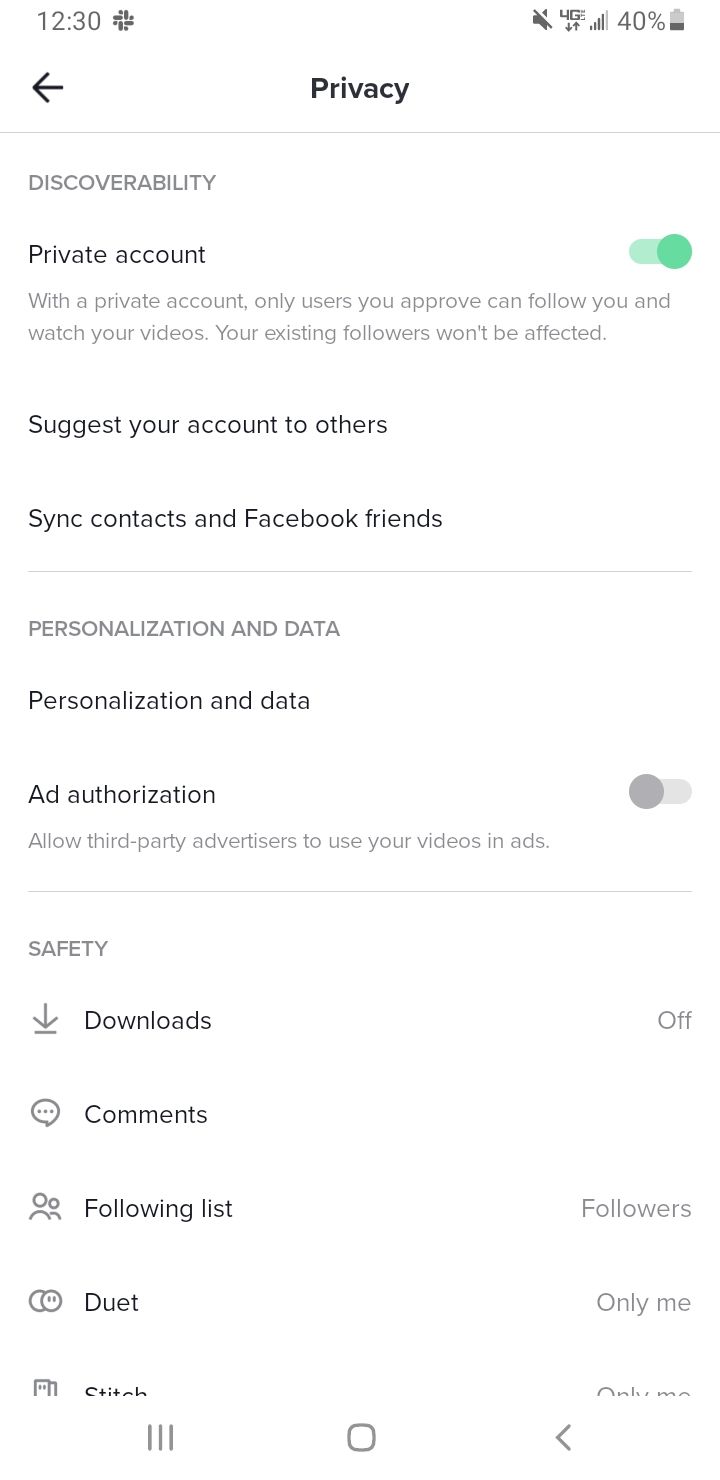In this image, we see a screenshot of a mobile device's settings. At the top left, the current time is displayed as 12:30. The top right corner reveals several status indicators: the device is on mute, the 4G signal is active, the network signal strength is 4 out of 5 bars, and the battery is at 40%. 

Below this, various texts and options are visible. Under privacy settings, the account discoverability is noted, with "private account" checked, meaning only approved users can follow the account. There is an option to suggest the account to others and to sync contacts and Facebook friends. 

In the "Personalization and Data" section, "Ad Authorization" is not checked, indicating that third-party advertisers are not allowed to use videos in ads. 

Lastly, other options available in the settings include safety features such as downloads, comments, following lists, duets, and stitches.